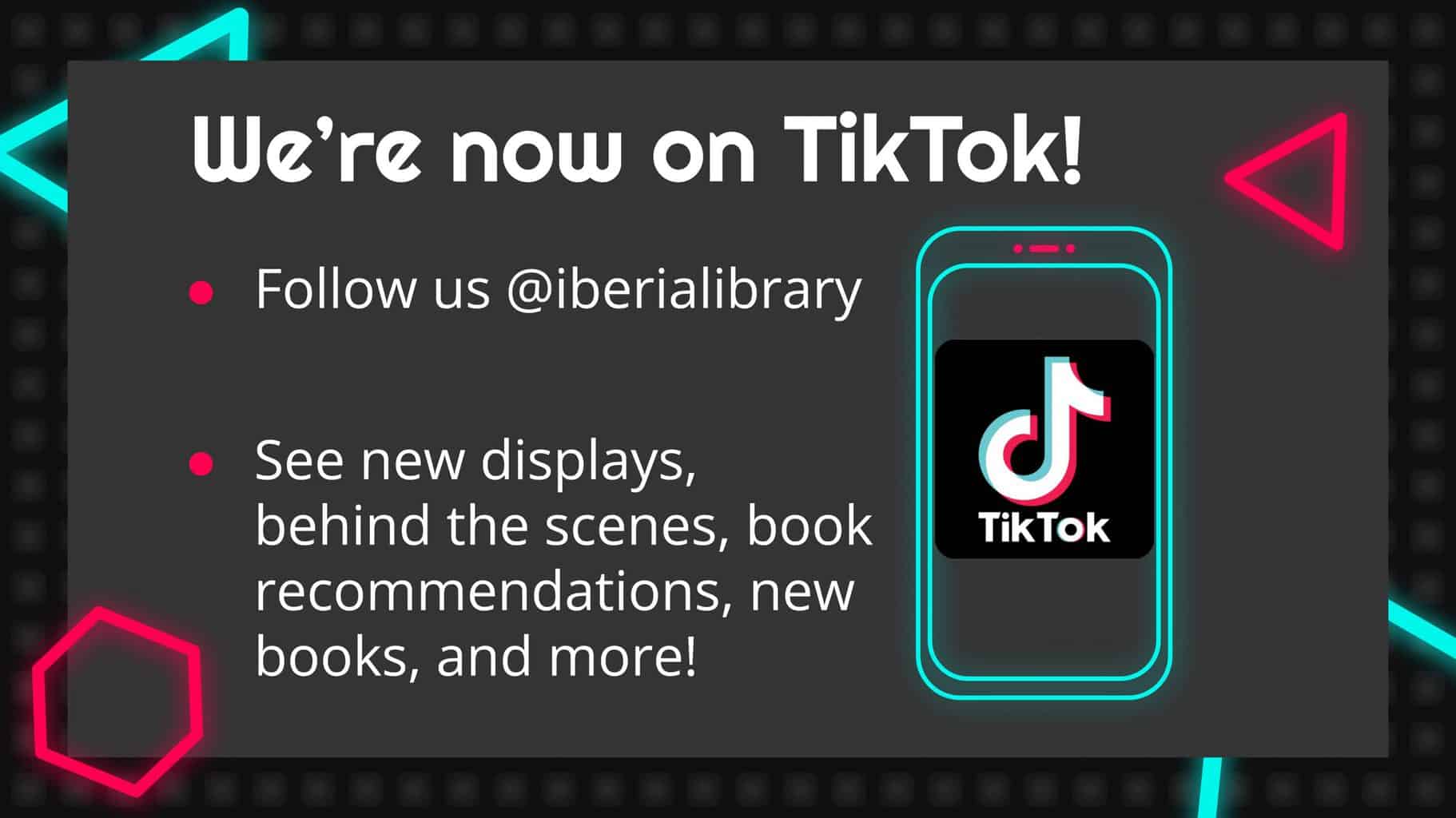Here is a detailed and cleaned-up descriptive caption for the image:

---

The screenshot from a webpage features an elaborate design set against a black background with numerous faded gray and white circles. Prominently displayed is a neon cyan blue triangle pointing to the left, juxtaposed with a hexagonal shape floating above a dark gray rectangle that stands out due to its red border. Adding to the visual complexity, a floating neon red triangle is also present.

To the right of the design, there is a silhouetted smartphone illustration composed of two rounded rectangles. The larger rectangle encases a smaller one, both outlined in neon cyan blue. The larger rectangle features two red circles and a neon red line between them, depicting buttons arranged horizontally at the top.

On either side of the visual elements, two neon blue lines extend from the corners, adding symmetry.

The focal point of the dark gray rectangle is bold white text that announces, "We're now on TikTok!" Below this proclamation, white text next to red bullet points provides further details:
- "Follow us at @iberialibrary"
- "See new displays, behind the scenes, book recommendations, new books, and more."

The overall aesthetic combines neon hues, geometric shapes, and informational text in a visually appealing and dynamic layout promoting the presence on TikTok.